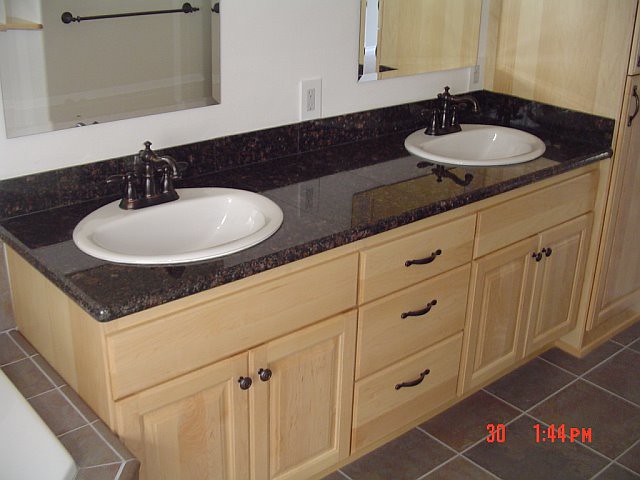The image depicts a pristine bathroom, captured in a time-dated snapshot at 1:44 PM on an unspecified day. The bathroom, which could be part of a newly constructed or recently remodeled home, appears immaculate and potentially staged for show.

The flooring features brown square tiles with light-colored grout, and this tiling extends to the base of a garden tub partially visible in the lower left corner of the photograph. The tub and floor share the same tile design, adding to the cohesive look of the space.

At the center of the image is a double sink vanity made of light-colored wood, possibly maple or another blonde wood variety. The vanity's countertop is striking with its black granite interspersed with copper flecks. A backsplash runs along the wall behind the sinks, with an additional sidesplash on the right where the vanity meets what seems to be a matching linen closet or stacked cabinetry.

Each sink, made of simple white porcelain in an oval design, is paired with an industrial-looking, oil-rubbed bronze center-mount faucet. These faucets are uniform in style across both sinks.

Above each sink hangs a beveled, unframed wall-mounted mirror, adding to the clean and modern aesthetic of the bathroom. Below the mirrors, there's a sleek, rectangular electrical outlet flush with the backsplash, providing a convenient yet unobtrusive power source.

The vanity’s cabinetry includes two false drawers under each sink, a set of three central drawers, and double doors beneath each sink, all adorned with oil-rubbed bronze pulls and knobs that match the faucets. 

A digital timestamp in orange letters is visible in the lower right corner of the image, displaying the numbers "30" and "1:44 PM." This detail suggests that the image might have been captured by a security camera or a digital camera with date and time functionalities. The entire scene suggests a freshly completed renovation or a new build, meticulously organized and ready for potential buyers.